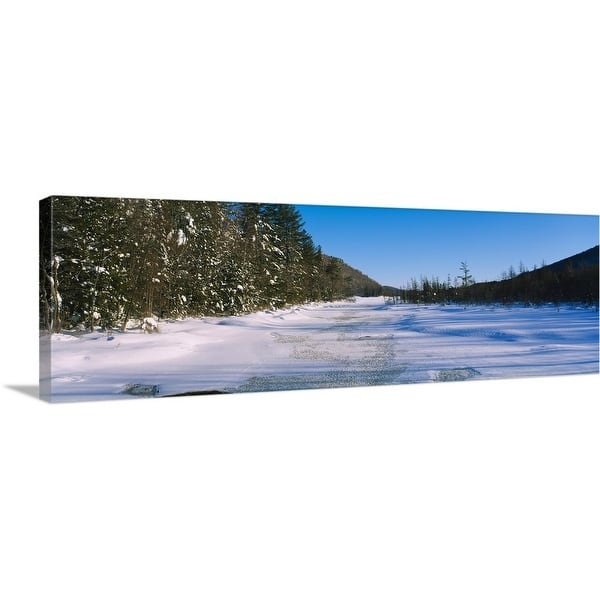This image shows a detailed photograph displayed on a printed canvas with the image wrapping around the sides, casting a noticeable shadow. The photo itself captures a serene, snowy landscape in nature. Dominating the foreground is a flat, snow-covered path, appearing to be a roadway with faint patches of asphalt visible beneath the thin layer of snow. This path stretches from the bottom and tapers off into the distance, creating a strong perspective effect. Flanking this path, there are clusters of green pine trees prominently on the left and right sides of the image. On the right side, the photo includes some scraggly, leafless trees extending towards the center, alongside a small hill dotted with additional green pine trees. Set against a backdrop of a clear, bright blue sky, devoid of clouds, this image captures the tranquility and natural beauty of a snowy forest pathway. No other background elements are present behind the canvas, highlighting the image against a clean, white screen.